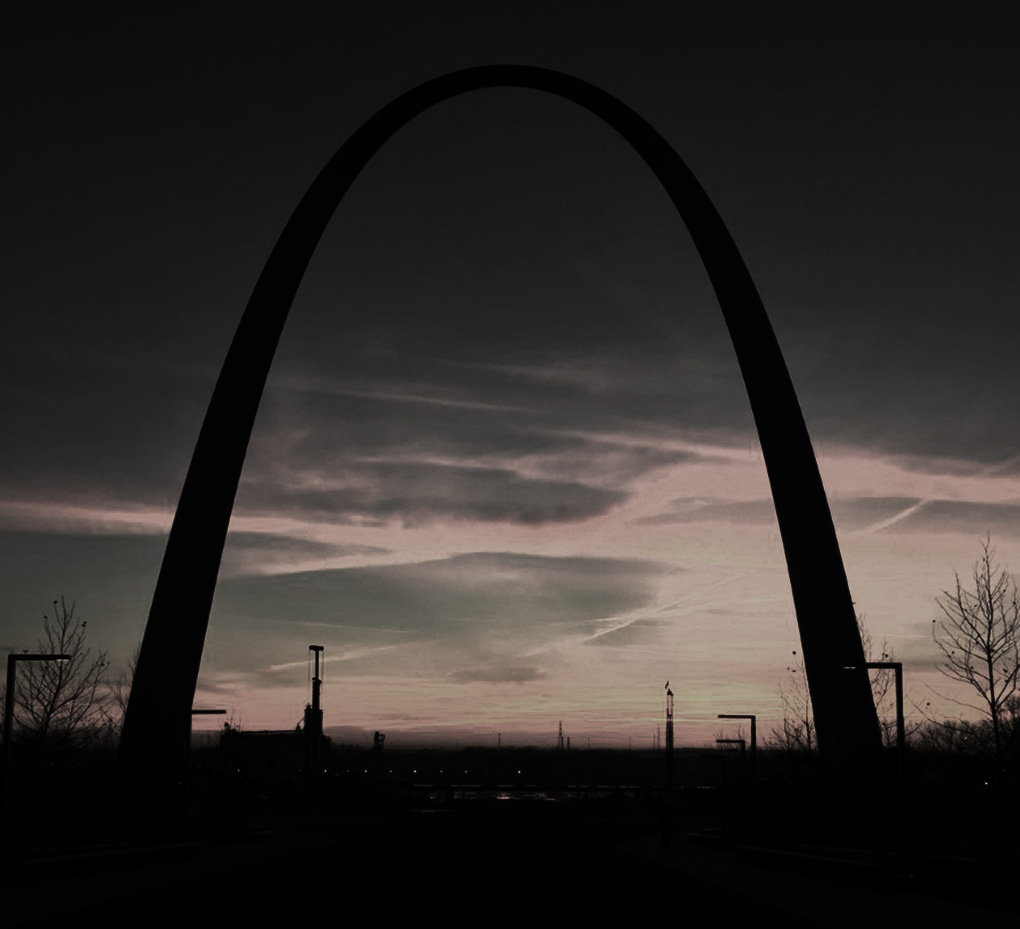The black and white image, captured during the transition from day to night, or perhaps early morning, is enveloped in darkness, with only a faint light remaining. Central to the scene is a large arch, resembling an overturned "U", dominating the composition. The right-hand side towards the lower half of the image is slightly brighter, suggesting the last remnants of daylight. The sky, barely visible, is streaked with faint pink, yellow, and off-white gray tones, with hints of blue against the overarching darkness. On both the left and right sides of the image, bare, leafless trees stand starkly against the dark background. Additional features include indistinct structures, possibly towers, and power lines that streak through the sky. The overall scene is engulfed in shadows, rendering most ground details obscure.